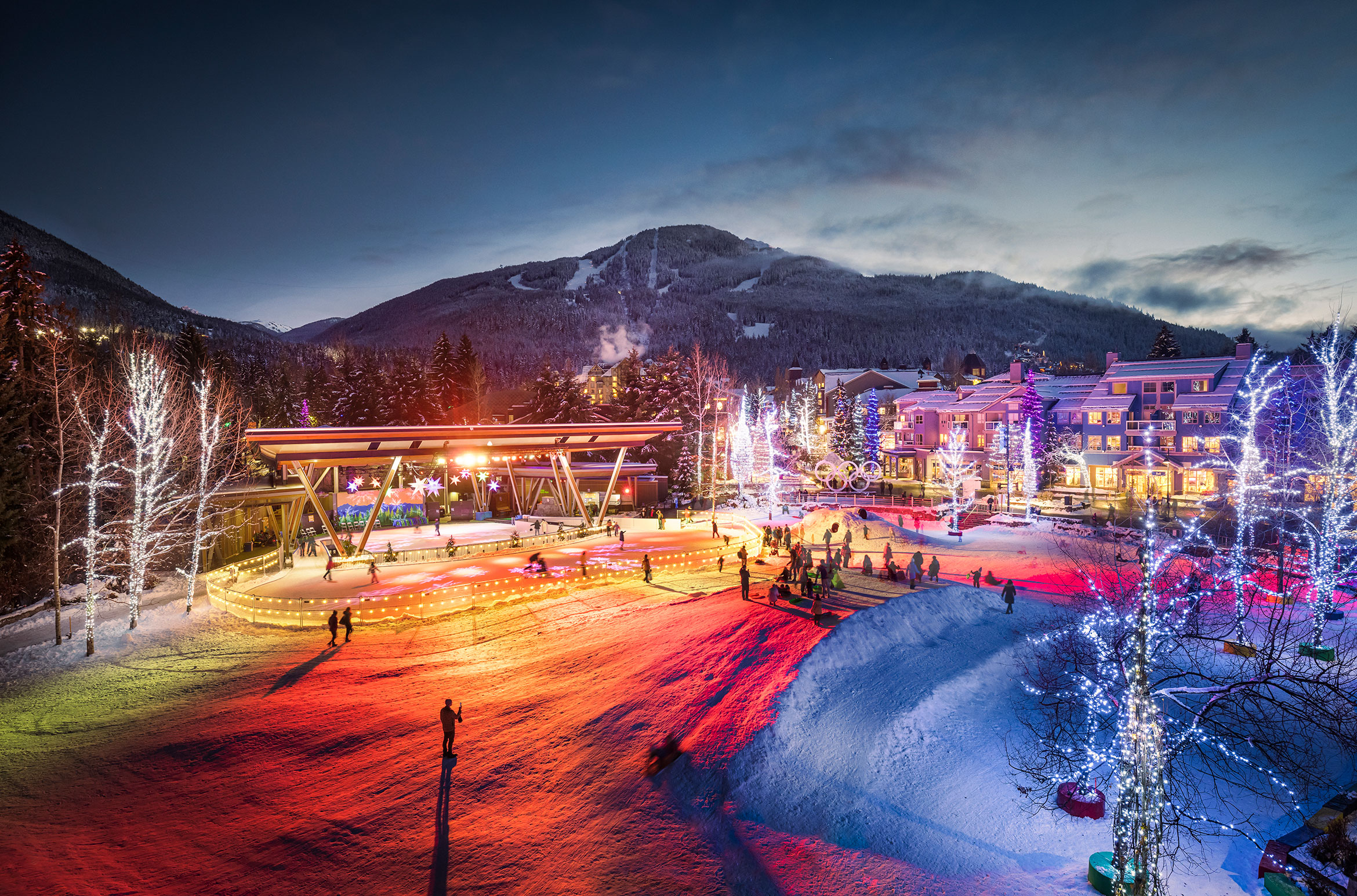This high-angle drone shot captures a vibrant and festive evening scene at an Olympic village in a snowy, mountainous region. The sky above is a contrast of deep blue in the upper left and grayish-blue in the upper right, dotted with clouds. The foreground reveals a bustling skating rink adorned with an array of bright and colorful lights, ranging from oranges and yellows to blues and reds, all reflecting off the pristine snow. On the left, dense clusters of pine trees, festooned with Christmas lights, add to the whimsical atmosphere.

In the distance, large, multicolored buildings reminiscent of ski lodges, one notably blue and another pinkish, create a picturesque backdrop. These buildings and trees are illuminated, casting a warm glow over the entire scene. The iconic Olympic logo is prominently displayed near a bustling square where visitors, not athletes, enjoy various entertainment options. The combination of the well-maintained snow, the lively crowd, and the radiant lighting make this scene a true winter spectacle.